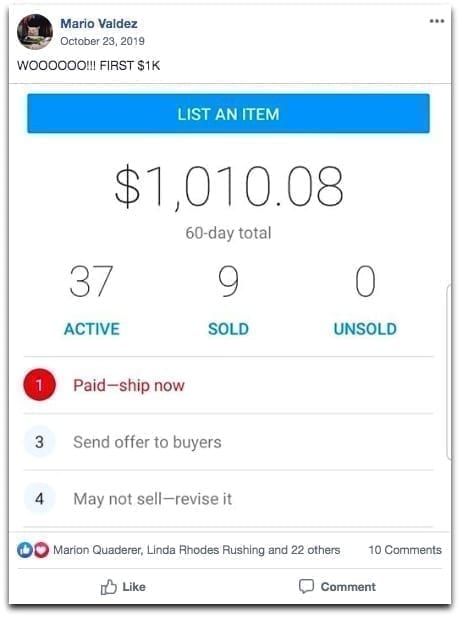The screenshot appears to be from a payment or e-commerce application, possibly reminiscent of Facebook in design. At the top of the screen, the user is identified as "Mario Valdez." The main highlighted text includes an enthusiastic note, "Woo! First 1K!" indicating an initial milestone achievement. The current balance displayed is $1,010.08, accumulated over a 60-day period.

Further details reveal that Mario seems to be selling items, as there is an option to "list an item." His activity summary shows 37 active listings, 9 sold items, and 0 unsold. Additionally, there is a numbered task list for transaction management which reads:

1. Paid
3. Ship now (needs attention)
4. Send offers to buyers
5. May not sell, revise it.

It appears that step 2 is missing, possibly due to an oversight or specific app design. The interface also shows engagement metrics with several people interacting with the post—evident by multiple likes—and 10 comments. The background of the interface is predominantly white.